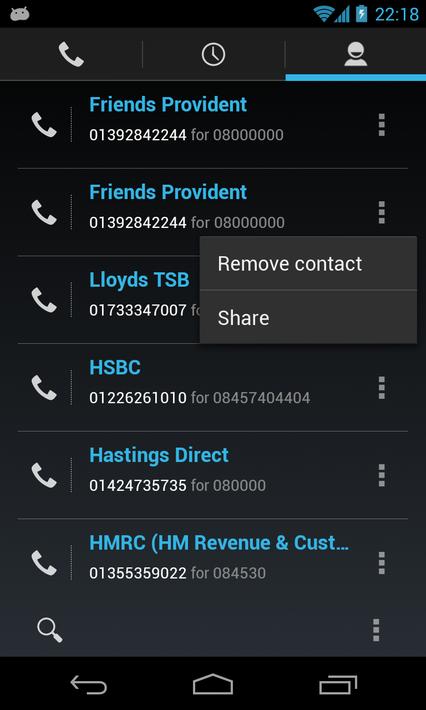In this image, a smartphone's contact application is displayed against a black background. At the top left corner of the screen, there's an icon depicting a phone call. Centrally positioned near the top is a recent calls icon, while at the top right, there's an icon for accessing the contacts list.

The contacts are listed below, with the contact names displayed in blue and the associated phone numbers in white. The first contact is labeled as "Friends Provident" with the phone number 01392842244, followed by the ambiguous sequence "408 and then the rest of the zeros." This contact is duplicated below with the same information and is currently selected, revealing options to either remove or share the contact.

Further down the list are additional contacts:
- "Lloyd CSB" with the number 013347007.
- "HSB" with the number 01226261010408457404404.
- "Hastings Direct" with the number 01424735735408000.
- "HMRC, HM Revenue and Customs" with the number 013553590224084530.

Each contact entry is flanked by a call button on the left and a vertical three-dot menu icon on the right, providing quick access to additional contact options and functions.